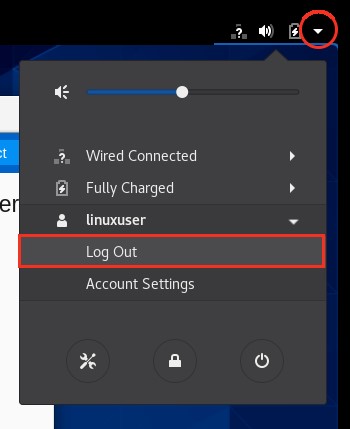The image depicts a user interface of a settings menu layered over a black background. The primary interface is set against a blue backdrop. On the left side of the interface, partially visible white text appears, although the words are cut off. A particular section is highlighted in blue.

Within the interface, there's a secondary section with a gray background featuring a control, possibly for adjusting light or volume, positioned slightly below the midpoint, indicated in blue. Below this control, the text "Wired connected" appears with a question mark icon and a white arrow adjacent to it. Further down, an image of a battery with a white lightning bolt is labeled "Fully charged," accompanied by another white arrow.

Next is the label "Linux user" with a downward-pointing white arrow and an adjacent white person icon. Below this, the term "Log out" is displayed in white text within a red box, indicating the log out option. A red circle surrounds another downward arrow icon at the very top. 

The bottom section of the interface lists "Account settings" in white text. At the very bottom, three distinct white icons are present: one resembling a wrench and screwdriver (suggestive of general settings or tools), another resembling a padlock (indicative of security settings), and the last one resembling a power button (suggestive of power options).